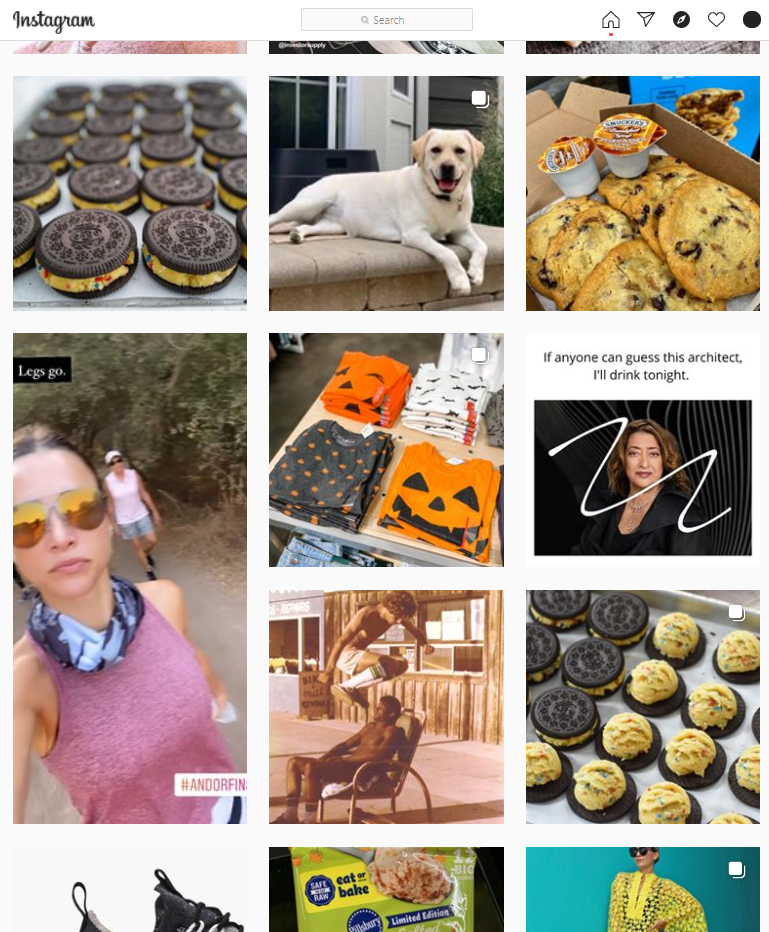The image showcases the Instagram Explore page viewed on a web platform. At the very top of the screen, the Instagram logo is located on the left-hand side, accompanied by a search bar in the center. On the right, there are five icons: Home, Share, Explore, Likes, and Profile.

The Explore section displays a variety of posts against a predominantly white background. The images and videos featured include:

1. A food-related image of cookies with filling.
2. A photograph of a Golden Labrador.
3. Another food image featuring more cookies.
4. Possibly a video of a woman.
5. An image displaying clothing items.
6. A meme.
7. A picture of a person sitting on a chair with someone else jumping over them.
8. A repeat appearance of the cookies, this time open-faced.

At the bottom of the screen, three more images are partially visible:
1. The first appears to be a shoe.
2. The second might be a snack.
3. The third shows someone wearing a dress.